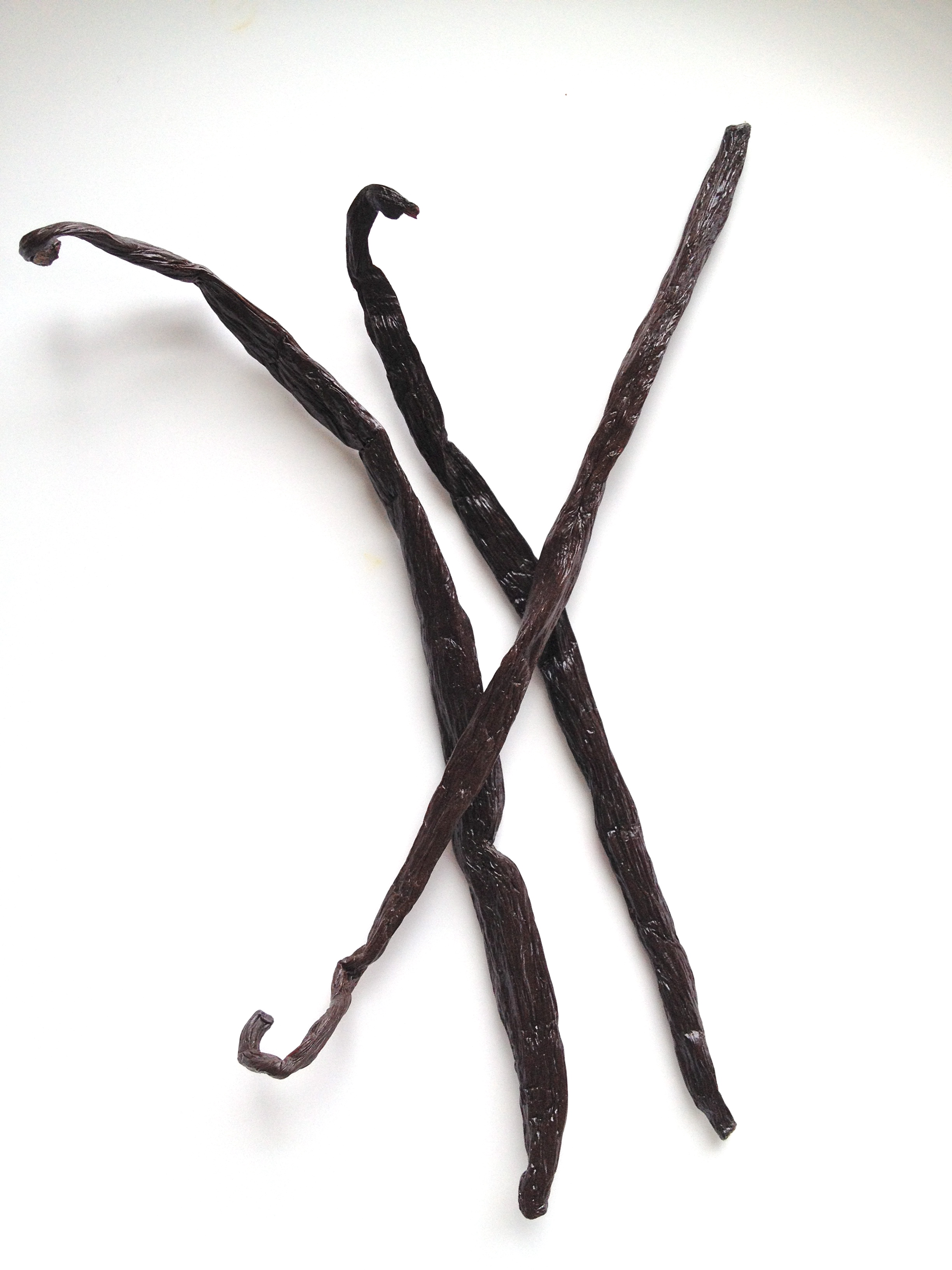The image shows three elongated, textured objects positioned on a predominantly white background with slight gray shading at the upper corners. The background itself is rectangular and vertically aligned. The objects, which appear to be either dried peppers, vanilla beans, or some other type of seed pods, are dark brown to nearly black in color and have a heavily crinkled surface texture. Two of these objects are placed side by side, diagonally stretching from the top left to the bottom right, while the third one crosses these two from the upper right to the lower left, creating a cross-hatched arrangement. The objects feature slightly curled ends, with the two parallel ones having their curled ends at the top and the crossing one having its curl at the bottom. Shadows beneath the curled ends add depth and contrast to the scene.